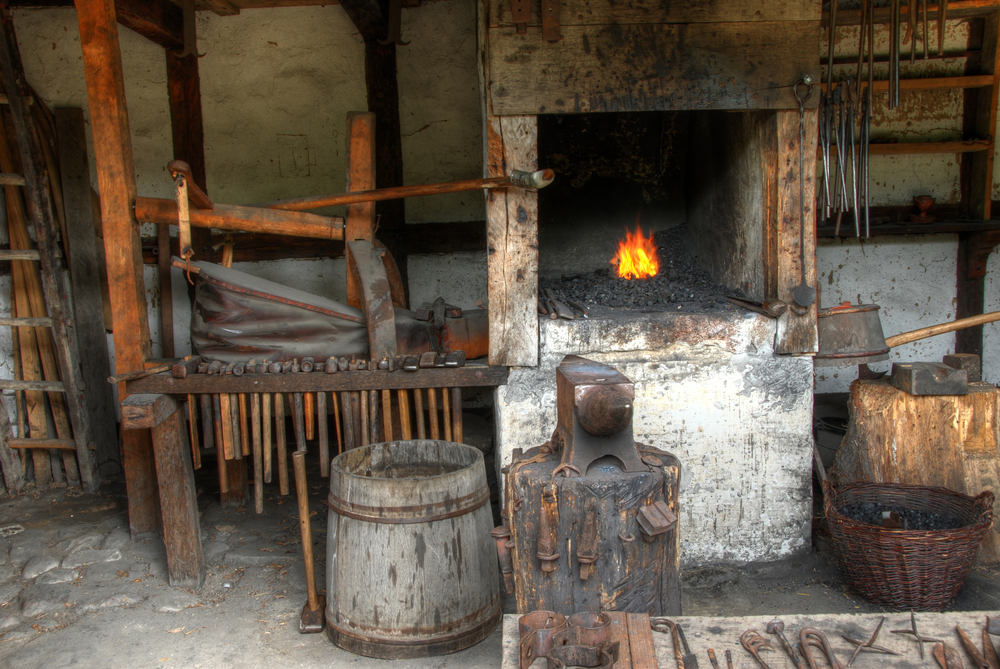The image depicts a detailed scene from a rustic blacksmith workshop, characterized by its medieval ambiance and various blacksmithing tools. At the heart of the workshop is a blazing furnace, or kiln, with orange-yellow flames illuminating the scene. In front of the furnace, there is a well-worn grayish-brown anvil seated on a cracked wooden tree stump, hinting at prolonged use. Surrounding the furnace, a variety of tools are organized: a large billow for fanning the fire, several hammers hanging from a wooden frame, and other blacksmith tools like prongs and tweezers, all showing signs of rust from continual exposure to intense heat.

To the right of the anvil is a dark brown wicker basket, sitting solidly on the gray stone floor, which is occasionally patched with concrete. On the left side, one can see a light brown, unfinished wooden barrel with a rusty hammer leaning against it. Nearby, there's likely a sledgehammer and other metallic shapes, possibly including hooks and shackles, scattered on an old wooden table cluttered with metal pieces of various forms.

The workspace is outdoors or semi-outdoors, suggested by the rustic wooden posts supporting the structure, painted dark brown with a reddish hue. The backdrop includes walls that seem to be made of plaster or concrete, adding to the aged and industrious feel of the workshop. The entire setting evokes a sense of history and craftsmanship, highlighting the blacksmith's dedication to their trade.